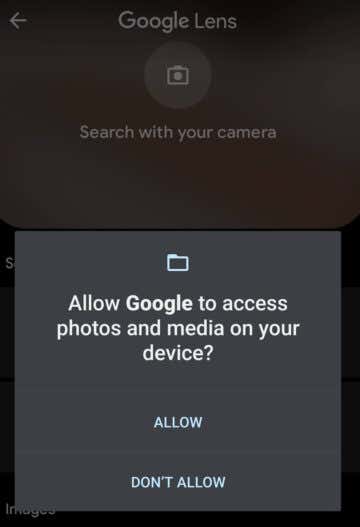This is a detailed screenshot of the Google Lens app on a smartphone. The app interface features a predominantly black background with grayish text. At the top left corner, there is a white left-facing arrow, and in the center of the top bar, the text "Google Lens" is displayed.

Directly below, there is a camera icon accompanied by the prompt "Search with your camera." Further down, a grayish box appears, containing a folder icon. The text within this box reads, "Allow Google to access photos and media on your device." Beneath this prompt are two options: an "Allow" link and a "Don't allow" link. Despite their appearance, these are links, not buttons.

In summary, this screenshot showcases the initial setup screen of the Google Lens app, instructing users to search using their camera and requesting permission to access photos and media stored on their device.